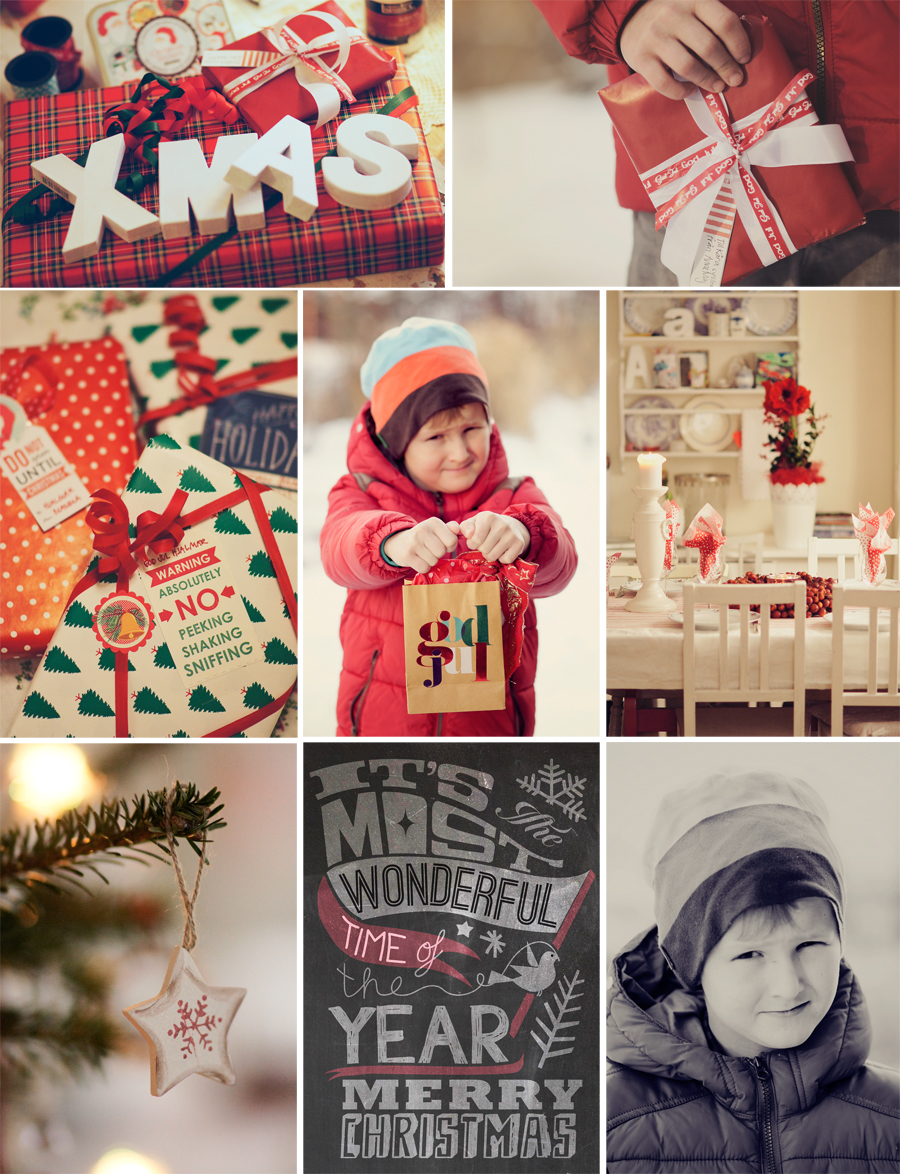This image is a vibrant Christmas-themed collage consisting of eight photographs arranged in a mixture of horizontal and vertical rectangles. In the top left, a partially cropped photo showcases a Christmas present wrapped in plaid paper with the word "XMAS" spelled out in letters on top. Adjacent to this, on the right, is an image of a small child dressed in a red coat and khaki pants, holding a red package tied with a bow. 

On the middle row, the first photo from the left features a gift wrapped in green Christmas tree paper with a red ribbon, bearing a tag that warns, "Absolutely no peeking, shaking, sniffing." Next to it, there is an image of a child in a hooded coat and beanie, presenting a gift bag with something visible inside. The background in this image is intentionally blurred. The final picture in this row displays a dinner table set up with silverware and dishes, and a shelf with numerous items can be seen in the blurry background.

The bottom row begins with a photograph of a Christmas tree branch adorned with a hanging star ornament, followed by a graphic with the message, "It's the most wonderful time of the year. Merry Christmas," on a dark gray background. The last image in the bottom right corner is a close-up, black-and-white photo of the child featured earlier.

The dominant colors in this holiday-themed collage are red and white, which unify the imagery and convey a festive atmosphere. This composition likely serves as an advertisement for gift wrapping, home decorations, or perhaps a store catalog or gift book cover, emphasizing the joyous preparations for Christmas.